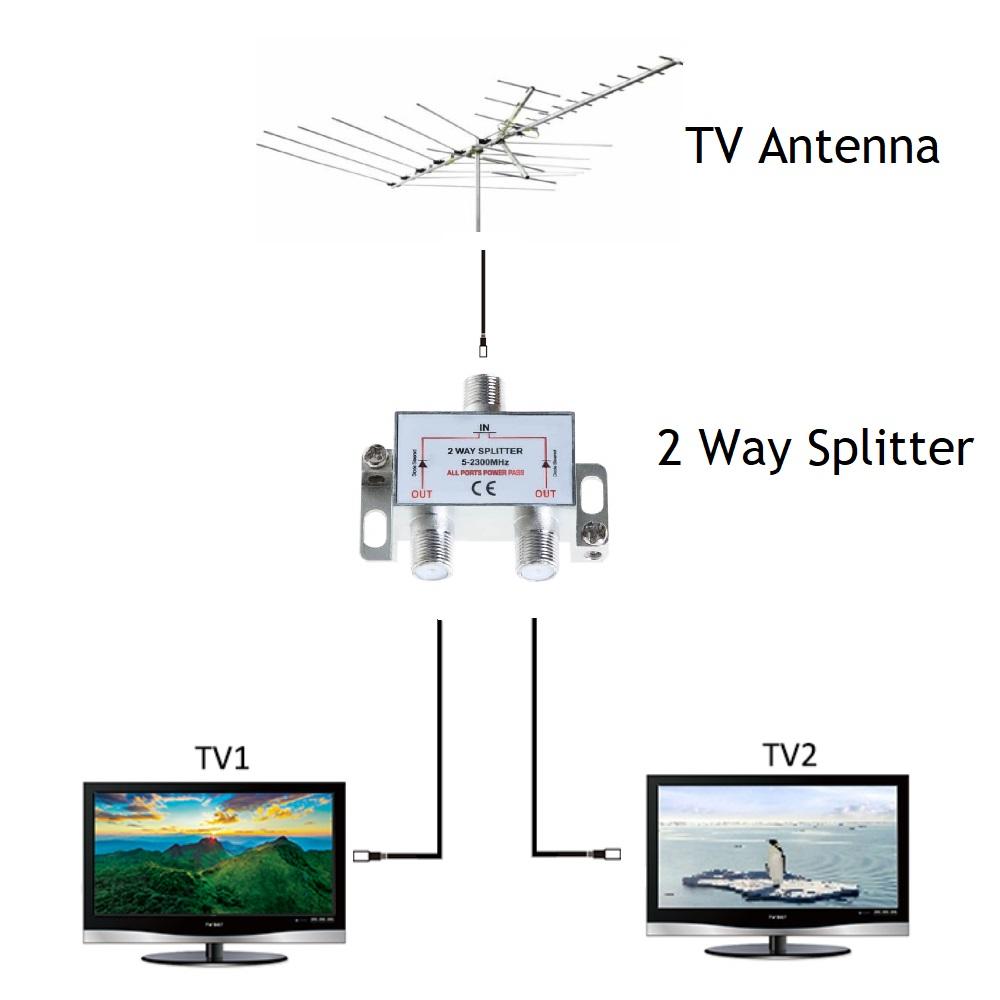The image is an informational schematic diagram with a solid white background, illustrating how to connect a TV antenna to two televisions. At the very top of the diagram, there is a black and white line drawing of a TV antenna, labeled "TV antenna." This antenna is connected by a cable to a metallic two-way splitter, which is also labeled "two-way splitter." 

From the two-way splitter, two cables extend downward. One cable leads to the left and connects to a small TV labeled "TV 1." This TV displays a scene of a green mountain range against a blue sky, indicative of a sunrise or sunset. The second cable extends downward to the right, connecting to another small TV labeled "TV 2," which shows an image featuring a penguin floating on ice.

The detailed elements include stylized circuit lines, shades of black, white, gray, and accents of light blue and red on the two-way splitter, and the distinct scenes displayed on each TV screen. The antennas are represented with multiple horizontal rods attached to a single primary rod, further enhancing the clarity of the connection process illustrated in the diagram.